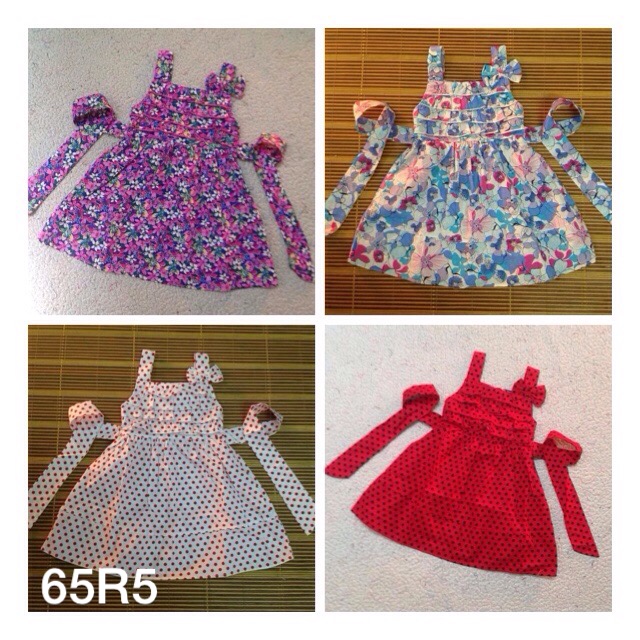This image is a collage of four photographs arranged in a square, each depicting a different dress with unique colors and designs, yet sharing a similar style. The upper left photograph shows a little girl's purple tank-style dress adorned with pink, white, and purple floral patterns, featuring ties on either side. Adjacent to it in the upper right corner, there's another dress with the same design but with a lighter background and larger flowers in blue, white, and pink. In the lower left, a white dress is dotted with black polka dots and laid out on the same light gray background seen previously. The final image, located in the lower right, depicts a red dress patterned with black polka dots, also showcasing ties on both sides. All of the dresses rest on either light gray or brown textured surfaces. Additionally, there are letters and numbers "65R5" visible in the lower left corner of the collage.